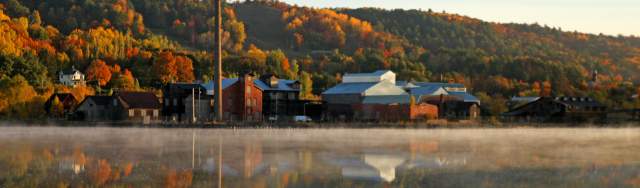The image depicts a narrow panoramic photograph of a quaint, rural town situated along a serene lakeshore. The townscape, nestled at the base of gently sloping, forested mountains, is dotted with large buildings characteristic of mid-20th-century architecture, suggesting a possible industrial past. Many of the structures are composed of red brick, wood, and gray stone, with sloping brown roofs, but one notable building with a white top stands out, its reflection prominently displayed in the mirror-like still waters of the lake below. This particular building, possibly a barn or a significant industrial structure, contrasts with the other dark red and brown rooftops of the town. 

The fall season is evident, as the surrounding trees exhibit vibrant hues of orange, yellow, and red, enhancing the picturesque quality of the scene. Soft mist lingers just above the water's surface, adding a ghostly, nostalgic aura to the otherwise clear reflections of the town's buildings, shoreline, and the vivid autumn foliage. Larger homes are scattered along the hills, peeking through the dense forest, which brings a warm, inviting atmosphere reminiscent of small Appalachian towns. The overall imagery captures a serene and picturesque autumnal setting, with the town's quiet charm reflected in the tranquil waters of the lake.